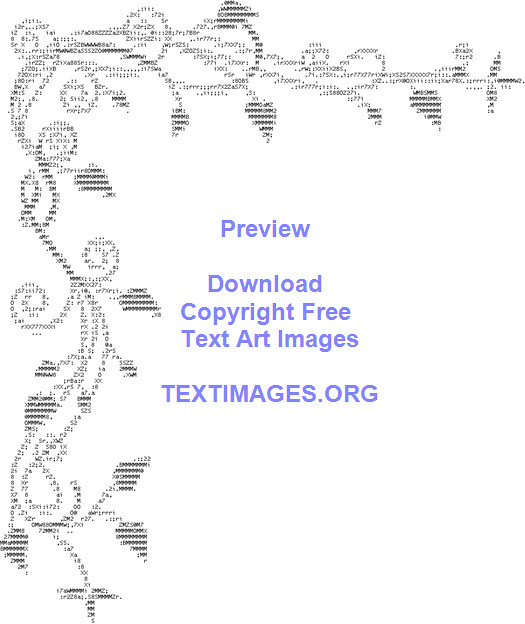The image features an intricate, detailed ring of flowers and vines composed entirely of text characters, symbols, and numbers, creating the appearance of leaves, blooms, and stems. These text-based elements, appearing black and strategically colored to simulate a natural floral design, journey from the upper right side, curve sharply to the left, and extend down to the bottom on a crisp white background. The leaves notably resemble the number 9. At the center of the image, in striking light purple text, the words "Preview. Download copyright-free text art images textimages.org" are prominently displayed. This gives the sense that it is an advertisement for the website textimages.org. The combination of the decorative text art and the clean, functional center text suggests a refined and creative representation, possibly designed by someone learning or demonstrating coding skills, reminiscent of HTML or CSS art.